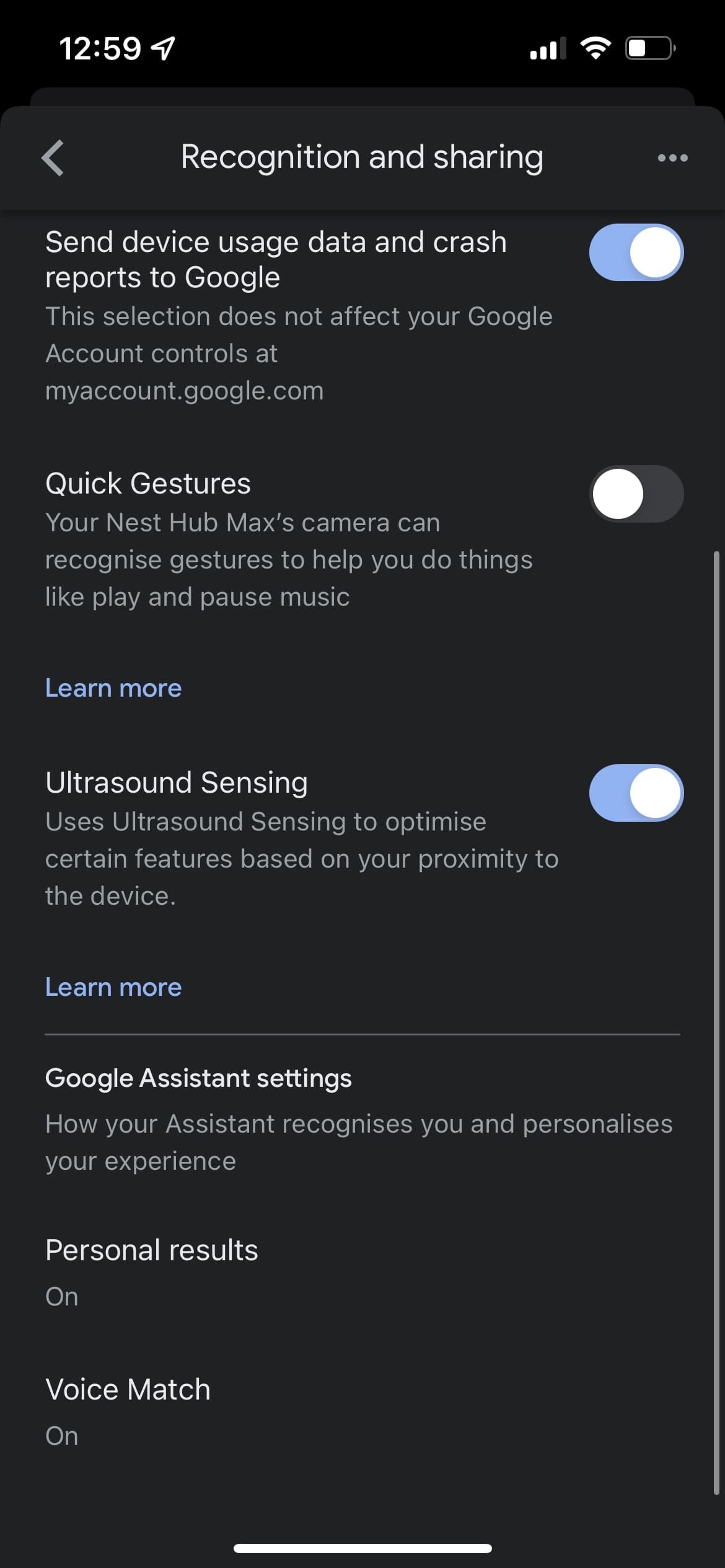The image shows a smartphone screen in portrait mode, displayed in dark mode. The background is predominantly black with white text. 

At the top left corner, the time is displayed as "12:59" alongside a small arrow pointing to the right. The top right corner displays the reception signal, Wi-Fi symbol, and a battery icon which is approximately 50% charged.

Right below the status bar, the following headings and options are visible:

1. **Recognition and Sharing**: 
   - An arrow pointing to the left accompanies this section. 
   - There are three dots on the right side which typically indicate more options.

2. **Send device usage data and crash reports to Google**:
   - Below this, in smaller gray text, it states: "This selection does not affect your Google account controls at myaccount.google.com".
   - On the right side, there is a blue toggle button which is in the 'On' position.

3. **Quick Gestures**:
   - Describes that the Nest Hub Max’s camera can recognize gestures to perform actions like playing or pausing music.
   - The accompanying toggle button for this feature is 'Off'.

4. **Ultrasound Sensing**:
   - Explains that ultrasound sensing is used to optimize certain features based on your proximity to the device.
   - The toggle button for this feature is blue and 'On'.
   - There is a "Learn more" link in blue text.

5. **Google Assistant Settings**:
   - In smaller gray text, it states: "How your Assistant recognizes you in person and personalizes your experience".

6. **Personal Results**:
   - Indicated to be 'On'.

7. **Voice Match**:
   - Also indicated to be 'On'.